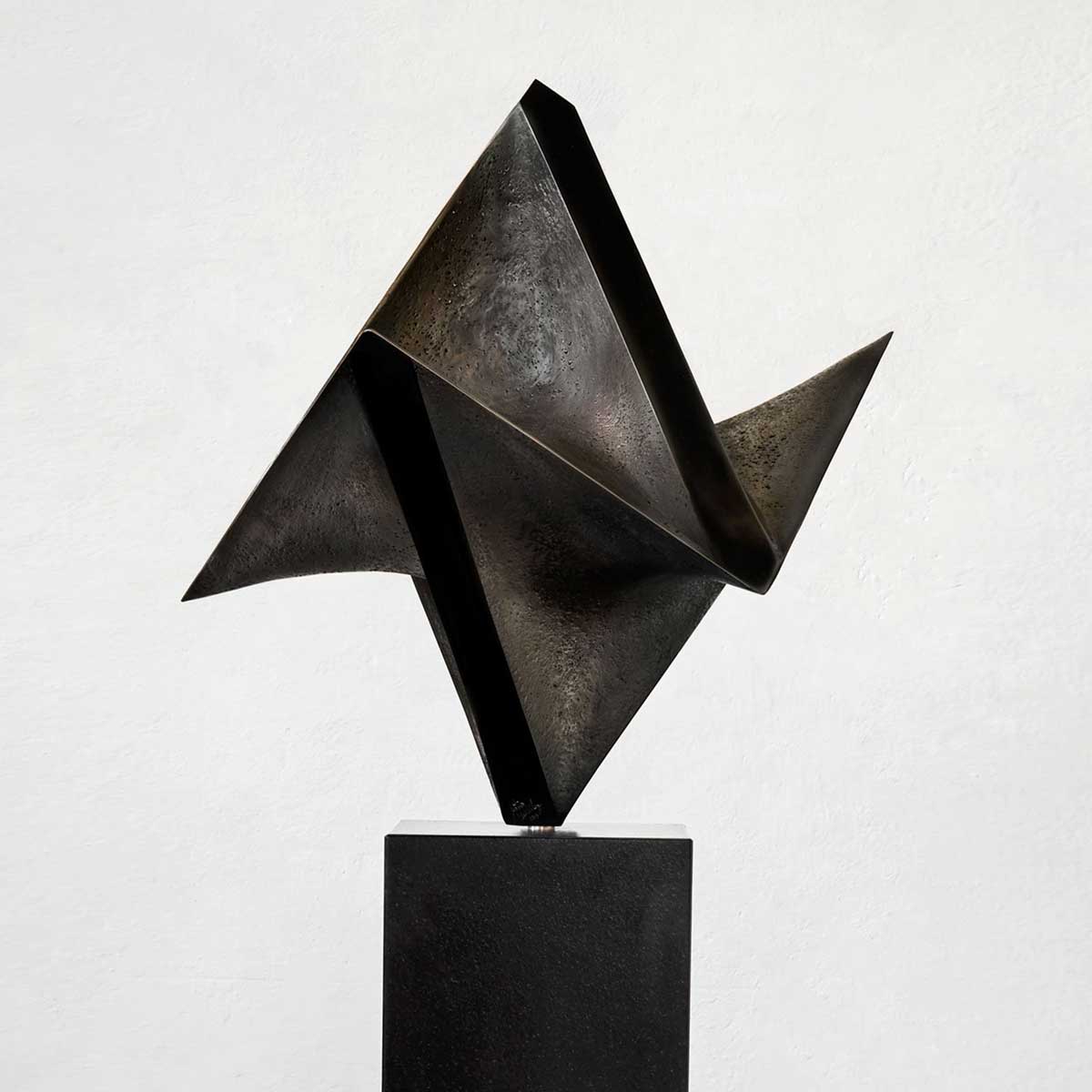This is a color photograph featuring an abstract, geometric metal sculpture, set against a white, slightly textured background. Constructed from dark metal, which appears to be a deep bronze or dark grey, the sculpture adopts an intricate design reminiscent of origami. It consists of folded triangular shapes, creating a complex form. Prominently, a large central triangle points upwards, flanked by additional triangles—one turned sideways at the bottom, with another pointing down on the left and one pointing up on the right. The sculpture's sharp, dynamic structure appears hollow inside and rests on a substantial black pedestal. The artist is not identified, and the photograph contains no people, animals, or other structures, leaving the focus solely on the striking metallic artwork.